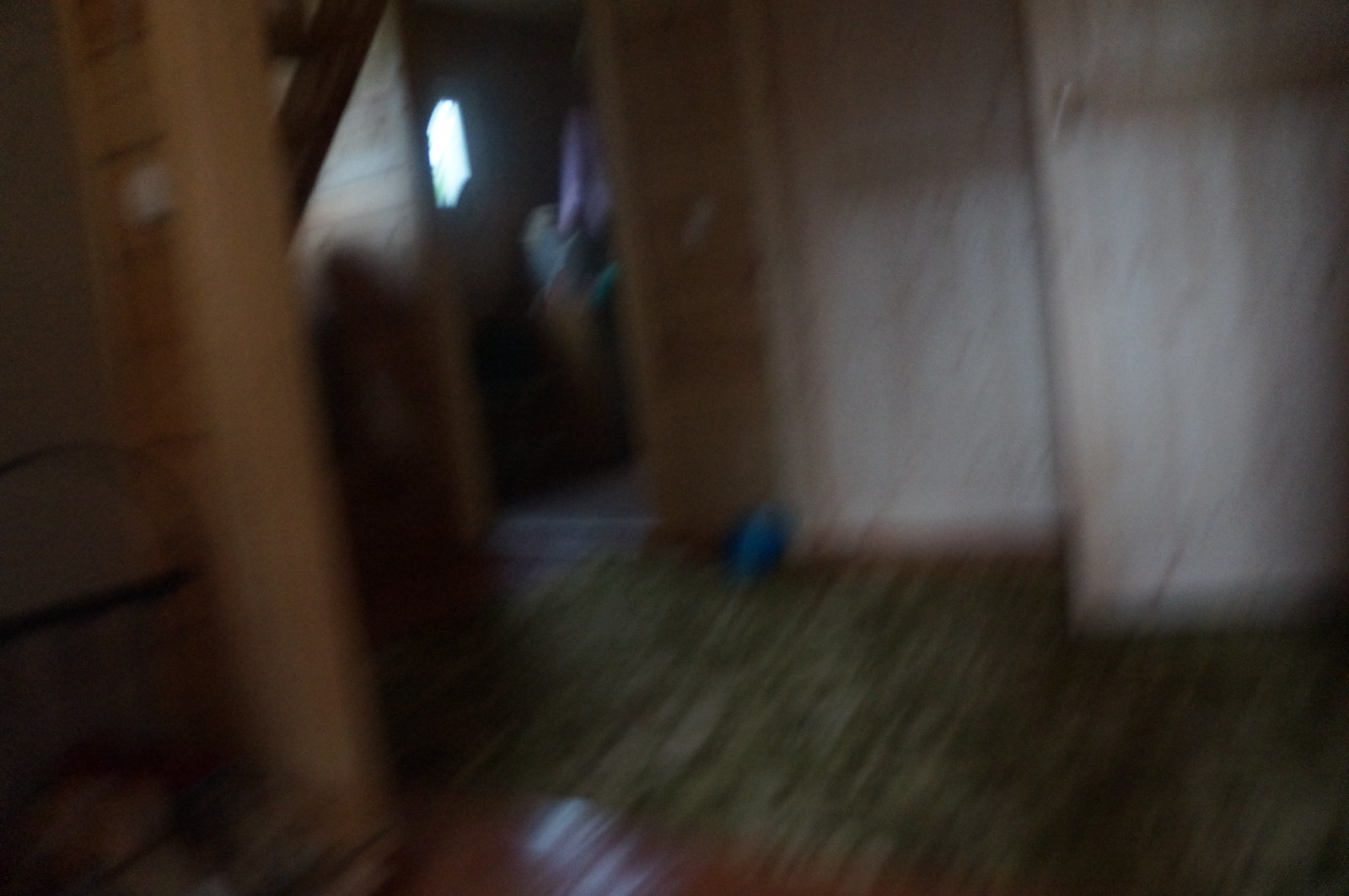This color photograph is blurry and out of focus with poor lighting, making it difficult to discern details clearly. Despite this, the floor appears to be a dark greenish-brown hardwood surface. In the upper right-hand corner of the image, two grayish-white doors stand open. Adjacent to these doors, there is a section of wall visible, painted a beige color. Beyond this wall, the photograph captures a glimpse of an adjacent room, illuminated by a small window, through which some light is streaming in.